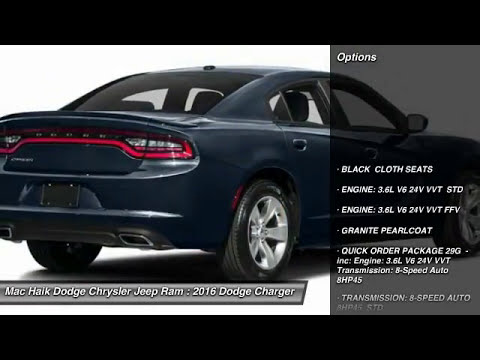The image appears to be a marketing material from a car dealership showcasing the back and passenger side of a dark blue 2016 Dodge Charger. The car is positioned at a 45-degree angle, with the front facing away from the viewer. Notable details include a red line area around the back lights and text at the bottom of the image reading "Mack Haik Dodge Chrysler Jeep Ram: 2016 Dodge Charger." On the right side, a partially translucent, shaded panel overlaps the car, displaying white text listing the vehicle's options: "Black cloth seats," "Engine 3.6 L V6 24V VVT STD," "Engine 3.6 L V6 24V VVT FFV," "Granite pearl coat," and "Quick order package 29G with engine 3.6 L V6 24V VVT, transmission 8-speed auto 8HP45." The words "Options" are prominently shown at the top of this panel, and the panel itself allows the car to be faintly visible through it. The image is framed by black bars at the top and bottom.